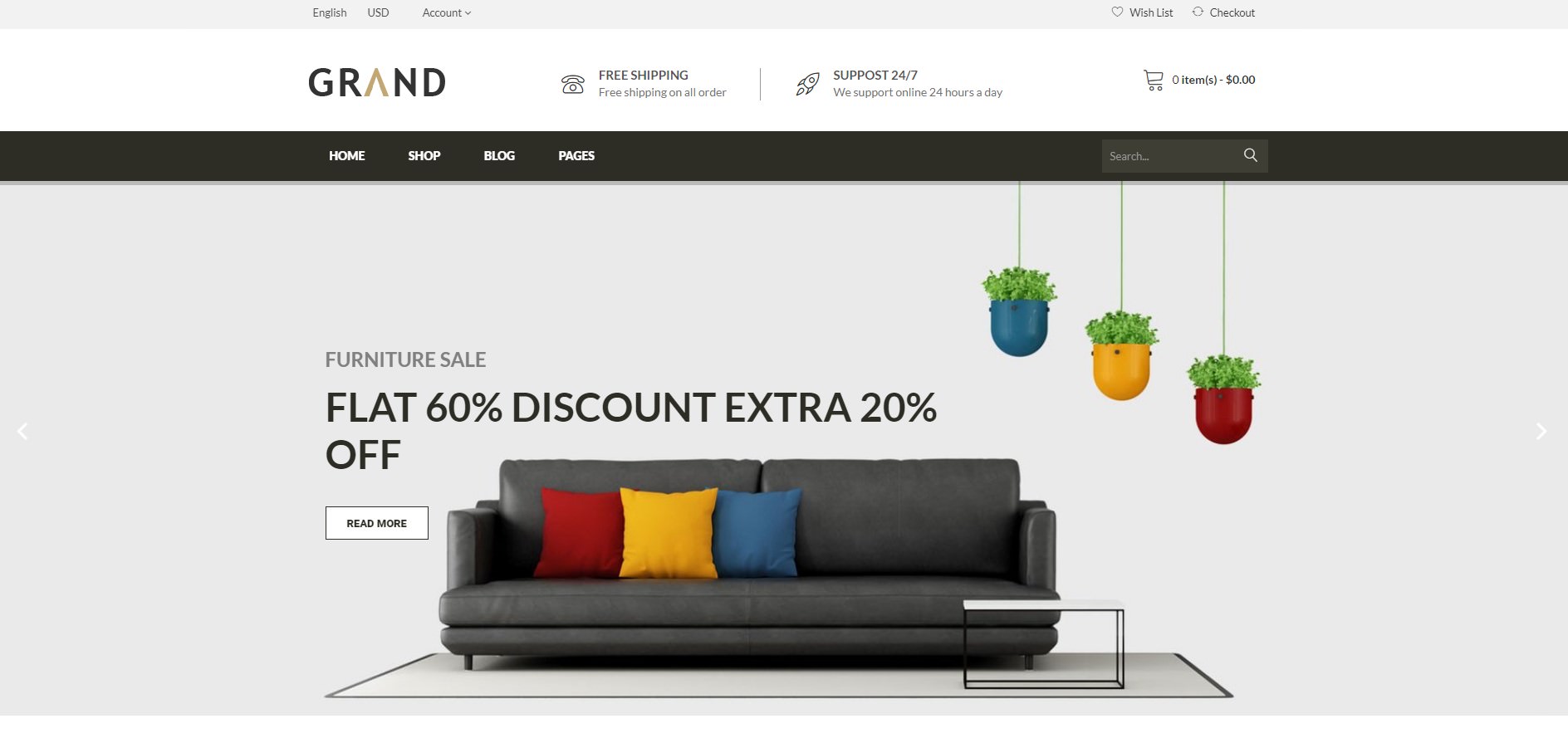The image features a clean, modern online furniture store interface. At the top, there is a small light blue box containing black text in English, USD, and other unspecified details, followed by a "Check Out" option on the right side. Below, a prominent white box displays the word "GRAND" in large black letters, with the letter 'A' in light brown. Next, a phone icon highlights benefits such as "Free Shipping" and "Support 24/7." 

Toward the top-right section, there is a shopping cart icon indicating a count of zero. Beneath this, a large black navigation bar with white text includes menu options: "Home," "Shop," "Blog," and "Pages," along with a search box for easy browsing.

The main background is light blue, showcasing a striking gray couch adorned with colorful red, yellow, and blue pillows. The couch rests on a light blue rug accented with a darker blue border. In front of the couch, there is a sleek coffee table featuring a white tabletop with black legs. Hanging from the ceiling are three vibrant plant pots colored blue, yellow, and red, each containing lush green plants.

Prominently displayed is a bold announcement for a "Furniture Sale" offering a flat 60% discount plus an extra 20% off. A white "Read More" button invites viewers to explore further.